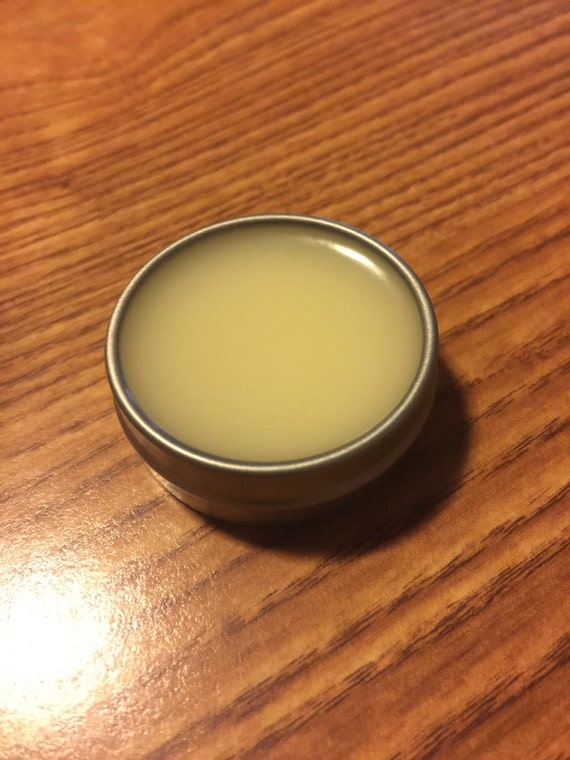This color photograph, presented in a portrait format, showcases a small, round metallic bowl holding a reflective yellow substance. This substance, smooth and shiny, suggests it could range from a gelatinous dessert like lemon curd to a waxy lip balm or even set candle wax. The bowl sits atop a medium brown, synthetic wooden table, characterized by its uniform grain and glossy finish. The lighting from the camera reflects off the table, creating a noticeable glare in the bottom left corner, while also accentuating the sleek, untouched surface of the yellow material inside the bowl. The bowl itself lacks a lid, emphasizing the pristine, unused state of its contents.